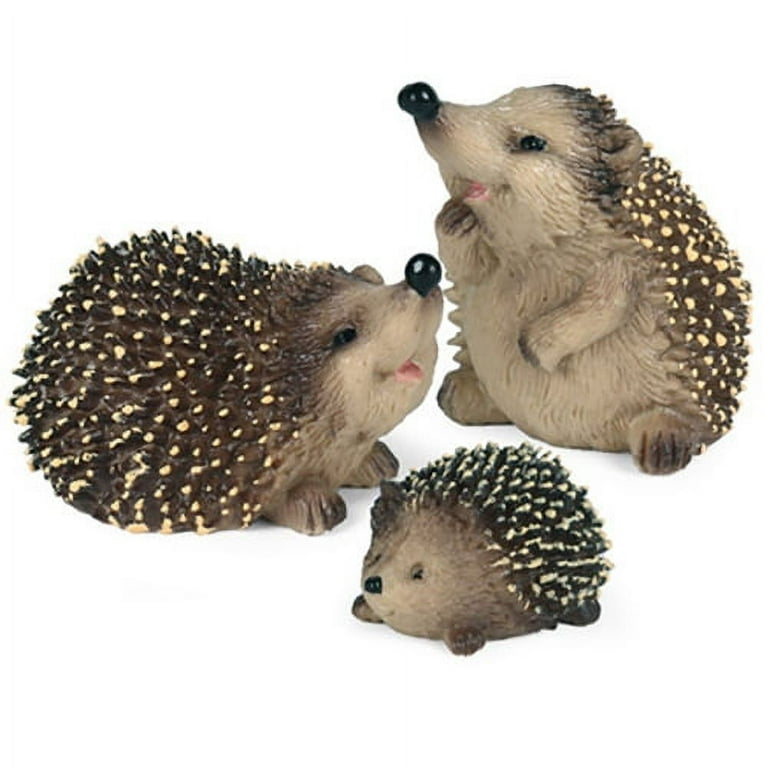The image features three highly detailed figurines of hedgehogs of varying sizes, meticulously crafted from what appears to be hardened clay, porcelain, or plastic. The smallest hedgehog, positioned in the foreground, has a light brown face and body, transitioning to darker brown with yellow-tipped quills. It is lying on its belly, smiling with a pink open mouth. To the left and slightly behind the smallest hedgehog is a larger figure, also smiling with an open mouth and pink tongue visible. This one is on all fours, looking upwards as if sniffing the air. The third and largest hedgehog is on the right, sitting on its hindquarters with its mouth open and seemingly scratching its chin. All three hedgehogs share a consistent color scheme: dark brown backs and light brown faces and bodies. The entire scene is set against a plain white background, giving the impression of a happy hedgehog family.